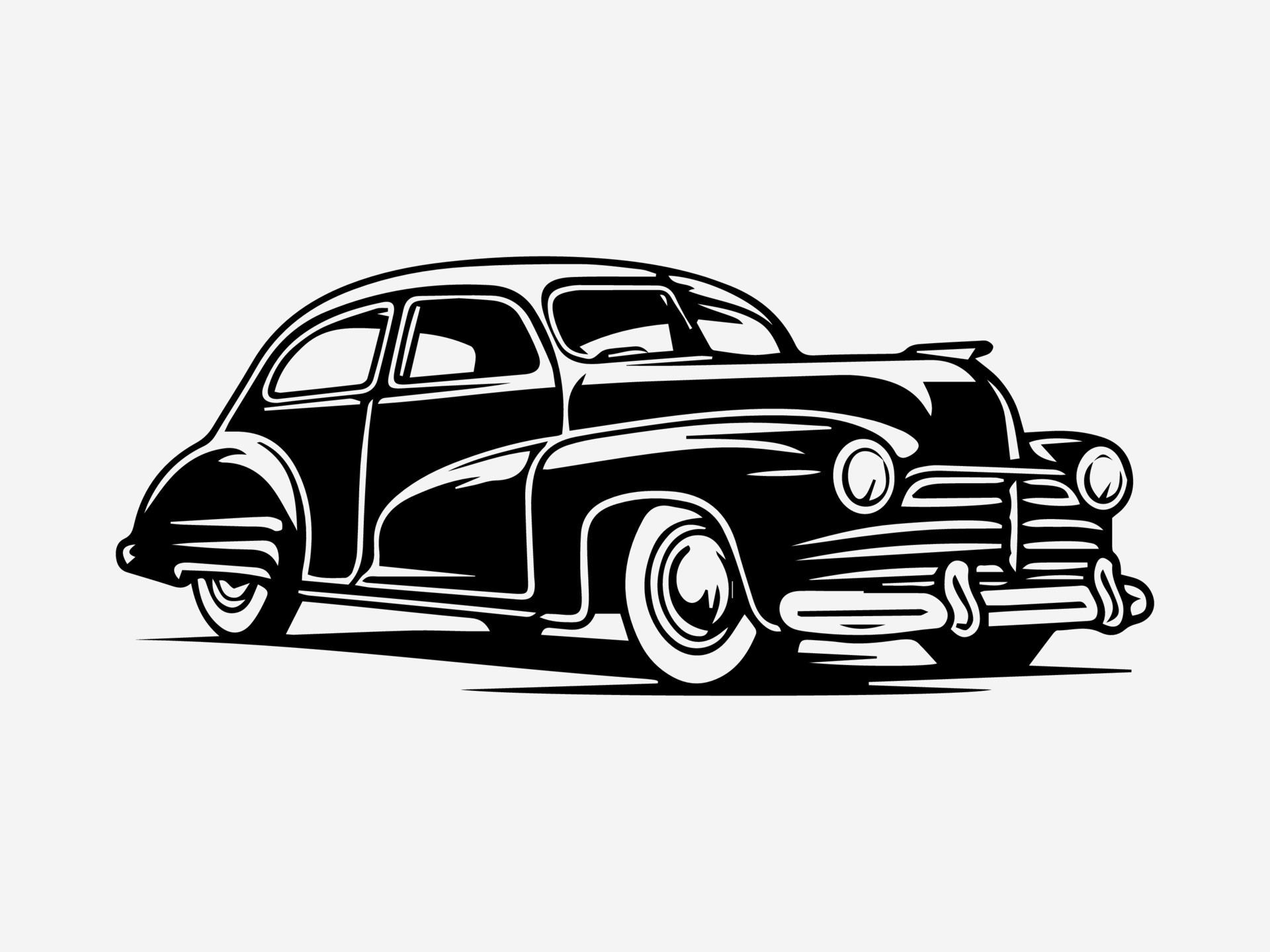This black and white artwork features a detailed illustration of a vintage car, likely a Studebaker, prominently centered against a plain white background. The car, facing right, showcases its long, thin hood, and a sleek body primarily in black with a contrasting white roof. It features two circular headlights flanking a silver grille and bumper. The vehicle has distinguishable white-walled tires with shiny metal hubcaps, and the rear wheel is partially obscured by a large fender adorned with three vertical white stripes. Notably, the car possesses a single side door, two side windows, and a wide windshield divided into two sections. The art also captures the car's shadow, adding to the depth and realism of the piece.